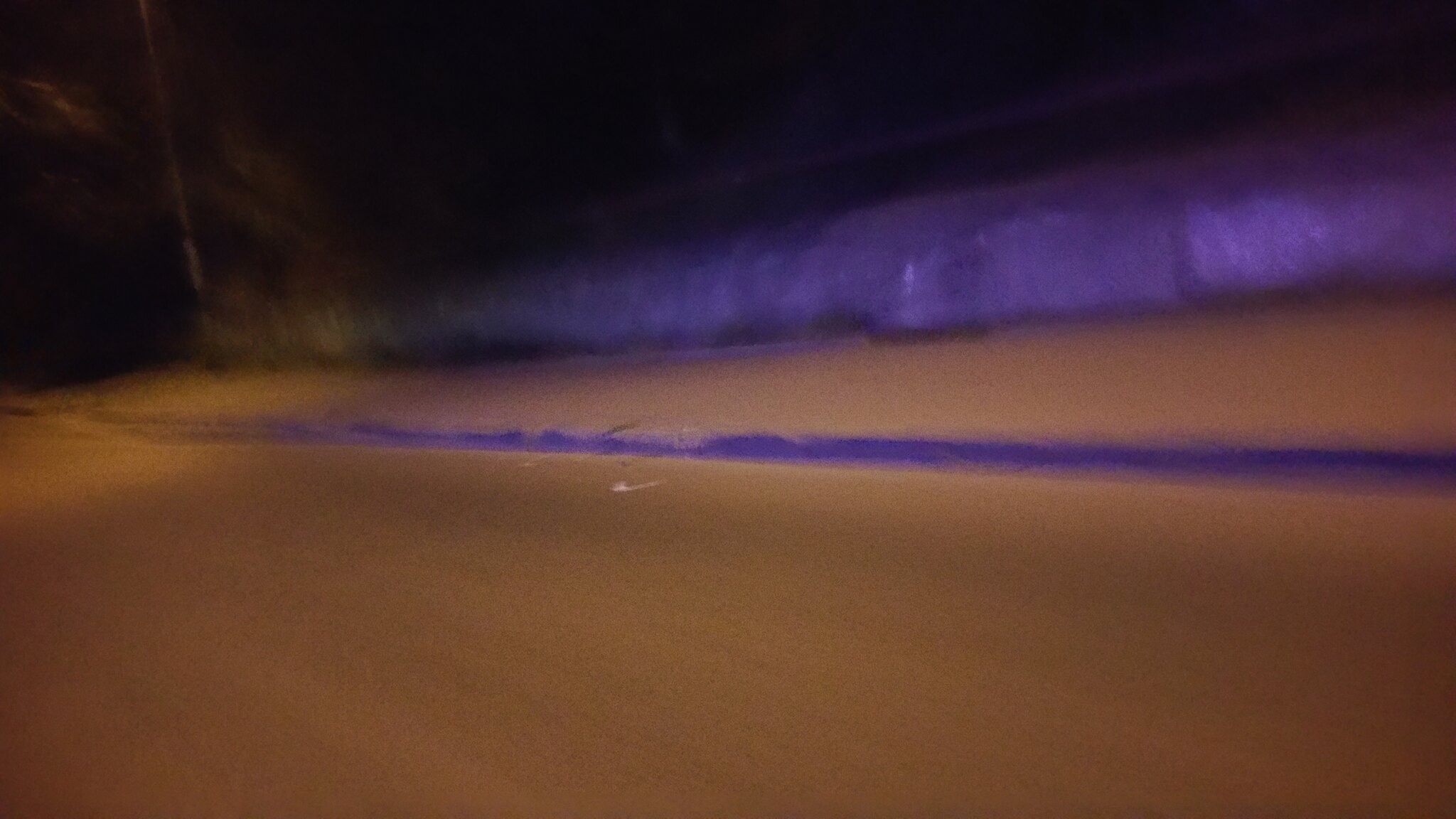This is an extremely blurry, low-quality photograph taken at night, likely from a moving vehicle. The photo displays a dark, solid black sky, indicating that it is quite late. The road itself appears tan-colored with a yellowish glow, possibly from street lighting, and is intermittently lit by blue and purple hues. A long purple stripe runs down the middle of the road, which might be made of fabric or plastic. To the left, the side of the road or possibly a bridge is visible with a cement railing and what seems like tall grass and bushes or a barrier covered in purple plastic. In the distance on the left, there are indistinct shapes, which could be trees and a pole. The overall blurriness and lack of focus make it challenging to clearly identify these elements.